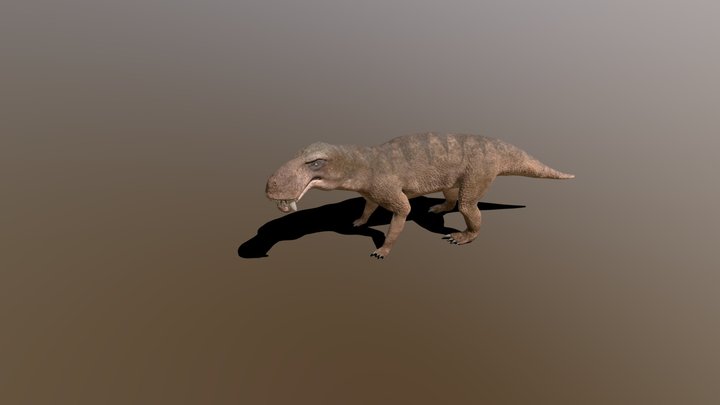The image depicts a digitally created, prehistoric dinosaur rendered from an angled overhead view. The dinosaur is primarily a mixture of light and dark browns, featuring distinct dark brown stripes running along its back. It stands on all four legs, which are somewhat short and stumpy, each ending with four sharp claws. The creature's tail extends straight out behind it, while its body casts a shadow on the ground to its left. This dinosaur has a long snout with two prominent long teeth jutting from its front, along with a visible yellow eye that appears deep and menacing. The background is a gradient from dark to light brown, starting darker in the bottom left and becoming lighter towards the top right, with the dinosaur centered amidst this backdrop. The texture of its skin is notably detailed on its back legs and stomach, adding a rich, realistic depth to the image.